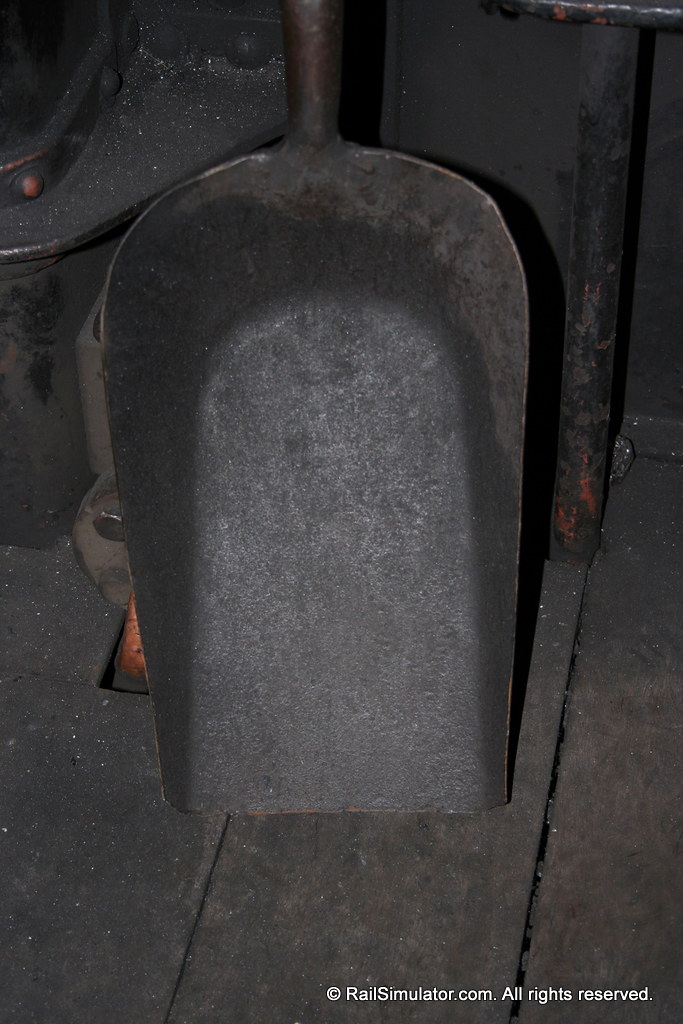The photograph captures a well-used coal shovel, resting on a wooden floor stained black with soot and ash. The scene is likely set within an old steam engine, possibly a museum exhibit. The shovel, predominantly black, shows signs of wear with chipped edges revealing the brown and gray metal beneath and exhibiting rust along the bottom edge. Only the lower part of the scoop and about an inch or two of the handle are visible. The shovel leans against a solid metal surface, dusted with ash and lightly marked with orange rust patches. Behind it, partial features of a metallic structure, likely part of the steam engine’s oven or stove, can be discerned. The photograph is marked with a white watermark at the bottom stating "railsimulator.com. All rights reserved."